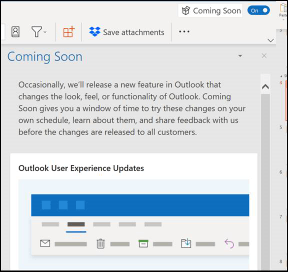The image is a partial screenshot capturing the upper right-hand corner of an Outlook interface. The background is gray, and at the very top, there is a menu bar containing several icons, including one for the account and another for saving attachments. In the top right corner, the text "Coming Soon" is displayed next to a blue, oval-shaped button labeled "On" in white. 

Beneath the header, the background shifts to light gray. In blue font, the text "Coming Soon" is repeated, followed by an explanatory paragraph: "Occasionally we will release a new feature in Outlook that changes the look, feel, or functionality of Outlook." 

At the very bottom of the screenshot, against a white background, there is a headline that reads "Outlook User Experience Updates." Directly below the headline, a blue line stretches horizontally across the image. The bottom section appears to contain some blotted out information, likely someone's account details.